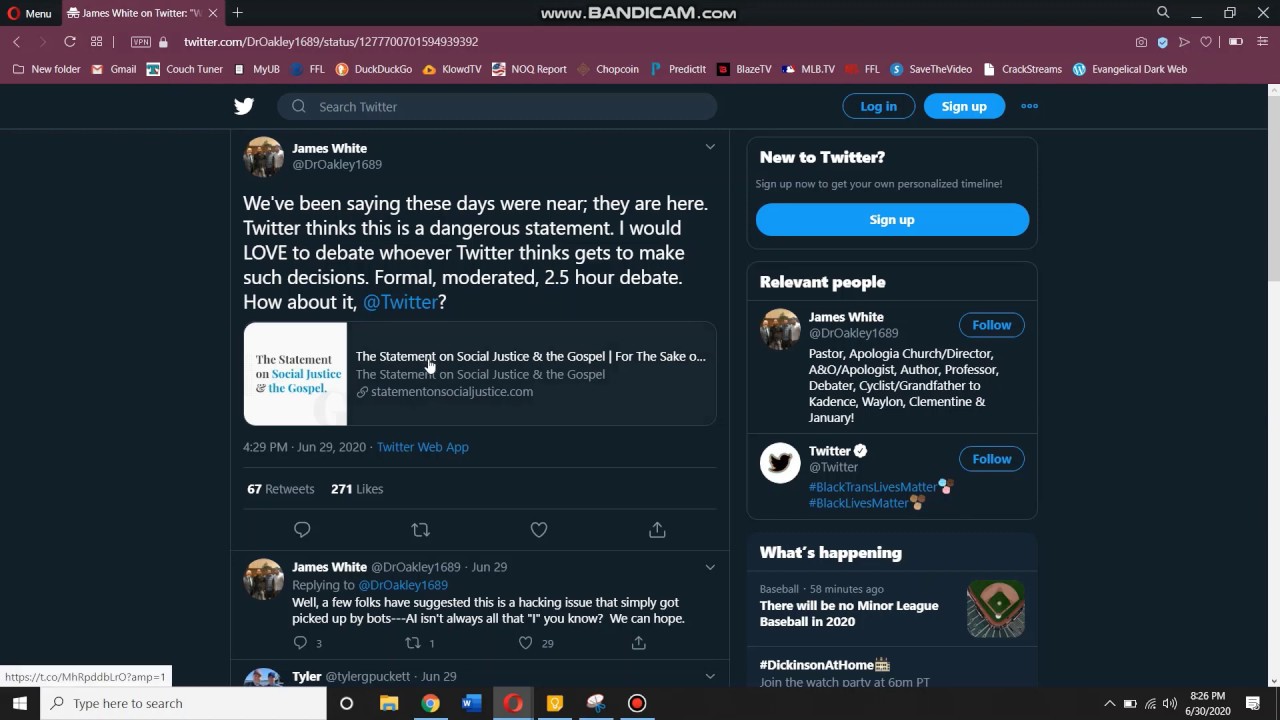The screenshot captured from www.bandicam.com features a Twitter webpage. In the upper left corner of the interface, the 'Menu' option is visible. At the top-center, the title bar from Bandicam indicates the screen recording tool used. The open window displays James White's Twitter profile, indicated by the text "James White on Twitter."

Below this, the URL in the web address bar reads "twitter.com/DrOakley1689/status/[number]." The screenshot prominently shows tweets, with two visible in the image. The top tweet, authored by James White, reads: "We've been saying these days we're near their hair. Twitter thinks this is a dangerous statement. I would love to debate whoever Twitter thinks gets to make such decisions. FOMO moderated 2.5 hour debate. How about it? @Twitter."

The second tweet, partially cut off at the bottom, is from Tyler Puckett and is dated June 29th. The visual context suggests the tweet stream is in mid-scroll, displaying ongoing activity from James White's Twitter account.

This detailed view provides insight into the specific interactions and statements made by James White, highlighting his challenge to Twitter's moderation policies.